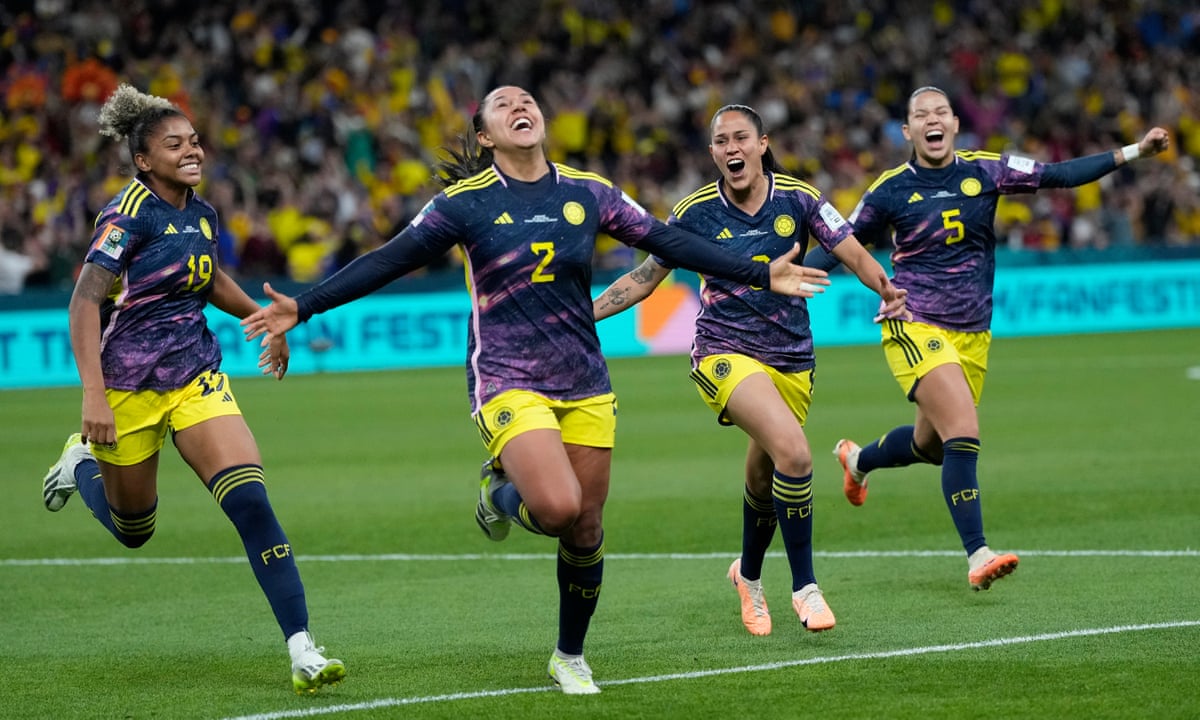The vibrant photograph captures a lively scene of four women celebrating triumphantly on a lush green soccer field, possibly after scoring a goal. The focus is sharply on the players, while the background blurs out a crowd of cheering spectators. The women are dressed in purple jerseys adorned with yellow stripes and numbers, with two wearing long sleeves under their jerseys. They sport yellow shorts featuring purple or blue stripes down the side, knee-high socks that are predominantly navy blue with yellow stripes and the letters "F.C.F." in front, and a mix of colorful cleats—some green, some orange. The image exudes joy and camaraderie as the players, identified by their numbers—19, 2, and 5—run with arms spread wide, celebrating their success on the beautifully maintained field bordered in blue.